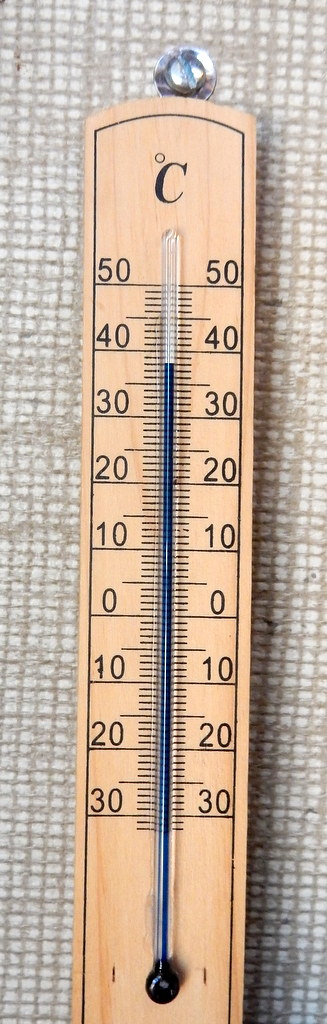A wooden thermometer is mounted on an exterior wall bathed in sunlight. The wall behind it features a pattern of small white squares with tan grout lines, adding a textured backdrop to the scene. A flathead silver metal screw secures the thermometer to this wall through a circular bracket at its top.

The thermometer, crafted from light-colored wood with a tan hue, measures approximately two inches in width. It is bordered by a thin black trim that runs along its sides, giving it a classic look. At the top, the thermometer displays a "°C" symbol indicating the scale is in Celsius.

The temperature scale on the thermometer ranges from -30°C to 50°C, with clear numerical markings for every ten-degree increment and smaller hash marks in between. At the center of the wooden frame lies a glass tube filled with a striking blue liquid, used to indicate the current temperature.